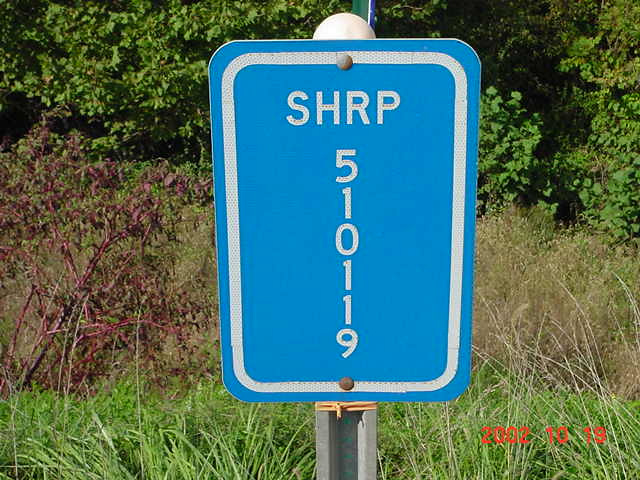This photograph features a road sign mounted on a silver steel pole, situated against a lush backdrop of green trees, tall grasses, and various shrubs. While most of the vegetation is vibrant green, there are patches where the foliage appears brown and dried out. In the bottom right-hand corner of the image, an orange date stamp reads "2002-1019." The road sign itself is a blue rectangle with a white border. At the top of the sign, in bold, white capital letters, is the acronym "SHRP." Below, arranged vertically from top to bottom in the same white font, are the numbers "510119."